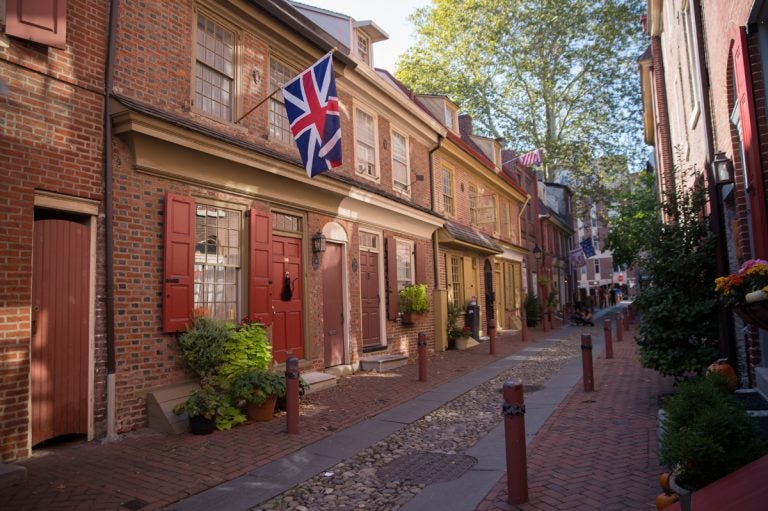The image depicts a charming residential street in Great Britain, characterized by its traditional architecture and quaint atmosphere. The focal point is a narrow stone path that runs through the center of the scene, flanked by numerous red metal poles. The path is bordered by brick sidewalks leading up to rows of attached townhomes on either side. Most of these homes are constructed from red brick, with some featuring lighter-colored bricks. The first home on the left stands out with its soft orange shutters and door, and prominently displays the British flag with its distinctive red, white, and blue colors. This home, along with two others, are two-story structures that contribute to the cozy, uniform look of the neighborhood. On the right side of the street, there is a large bush partially obscuring the view of additional houses. The background is adorned with lush greenery, including trees and house plants, adding to the scene's picturesque and serene quality. The image is devoid of text and people, offering an unobstructed view of this idyllic British residential street.